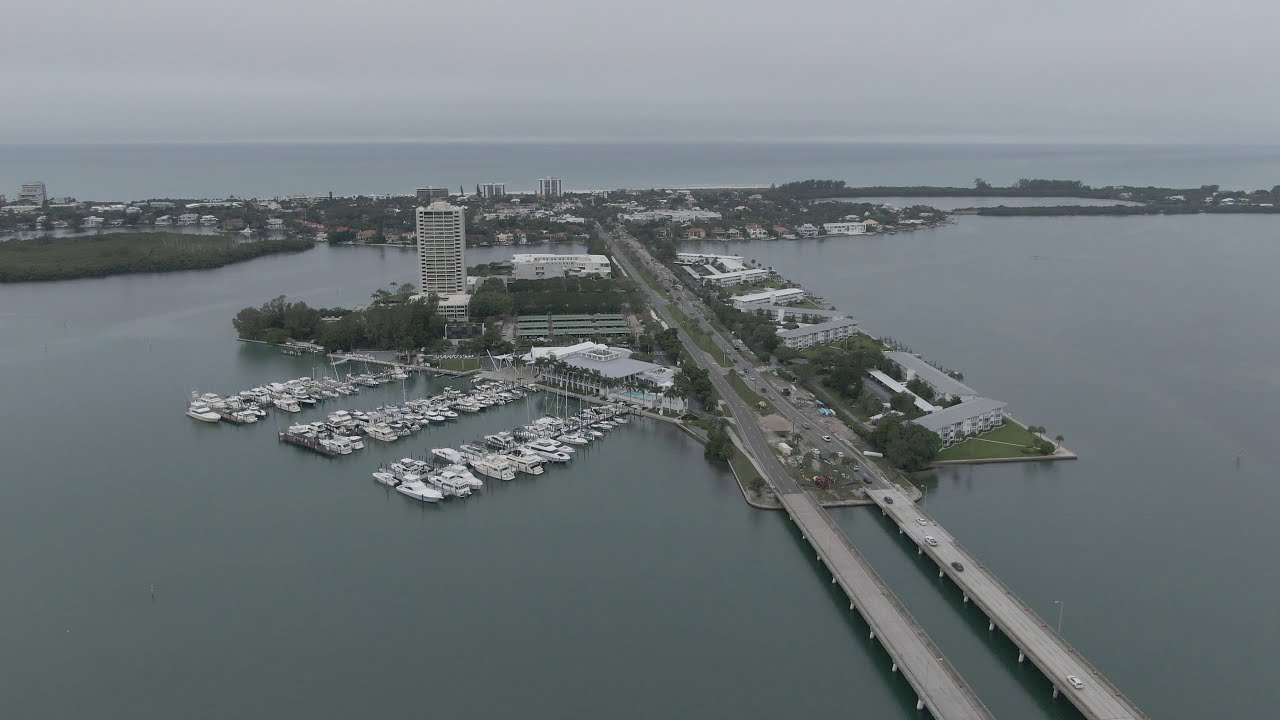The image presents an aerial view of a city that seems to be situated on or near an island, surrounded by an expansive body of water, possibly a sea or ocean. In the lower right-hand corner of the image, a four-lane highway bridge spans across the water, with cars driving on it. To the left of the bridge, three rows of stationary boats dock at three different docks, giving it the appearance of a marina. Behind this marina area, there is a mixture of buildings, including what appears to be a small skyscraper or high-rise, possibly a motel, surrounded by greenery consisting of trees and grass.

In the far right, the image features a circular area of water encircled by a coastline dotted with trees. Further to the left of this water circle are more land areas with various buildings and more greenery. In the far left-hand corner, another green patchy area with buildings is visible. The scene extends into the distance where the water merges with the horizon under a clear blue sky. Overall, the image portrays a city characterized by its blend of water, infrastructure, and natural greenery, suggesting a vibrant yet serene island cityscape.